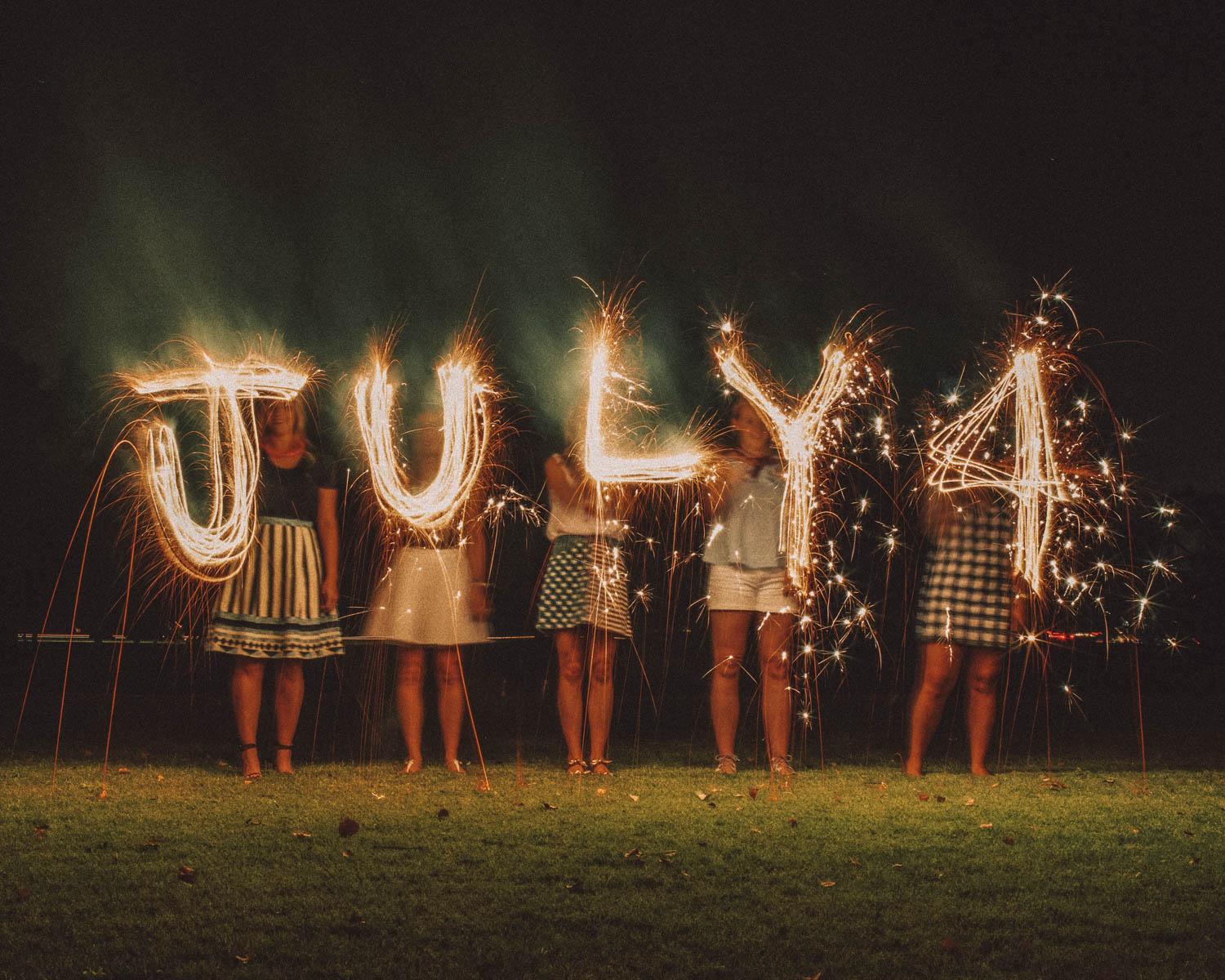This nighttime photograph captures a group of five women standing in a row on a grassy surface under a black sky. They each hold a glowing letter or number, spelling out "July 4" from left to right. The letters and number appear to be made of illuminated strings or wires, resembling sparklers. The J, U, L, and Y are followed by the digit 4. All the women are wearing skirts or shorts, and one, who is wearing shorts, has dark hair draping over her shoulder. The glowing letters cast a faint light on the grass below them, highlighting their immediate surroundings. The image composition is square, with the glowing characters spanning nearly the entire width of the image, positioned centrally. The setting suggests an outdoor nighttime environment, perhaps a backyard or park. The predominant colors in the image are black (sky), white (letters/numbers), and various shades of yellow, green, blue, and tan.